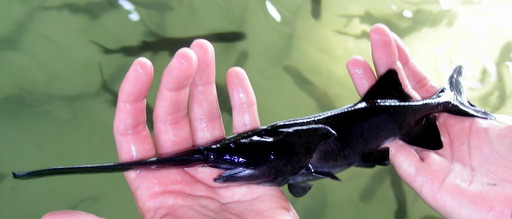In this detailed photograph, two hands, appearing to be of a white person, are carefully holding a small, delicate fish. The fish resembles a juvenile swordfish with its distinct, elongated, and somewhat wrinkled nose that spans nearly a third to half of its body length. Its body is mainly black, with notable features including black fins, a bluish underbelly, and a bluish mouth, which is open. The scene suggests the fish was freshly taken from a large, murky-green aquarium tank or rehabilitation center, evidenced by the other fish swimming in the background and the presence of rocks at the bottom. The light illuminating from the right side of the image highlights the fish's shiny, reflective surface and the wetness of the holder's palms. Interestingly, this peculiar fish lacks the typical side teeth on its extended nose, adding to its unique appearance. This content-rich setting provides an intriguing snapshot, possibly documenting an uncommon or newly observed species.